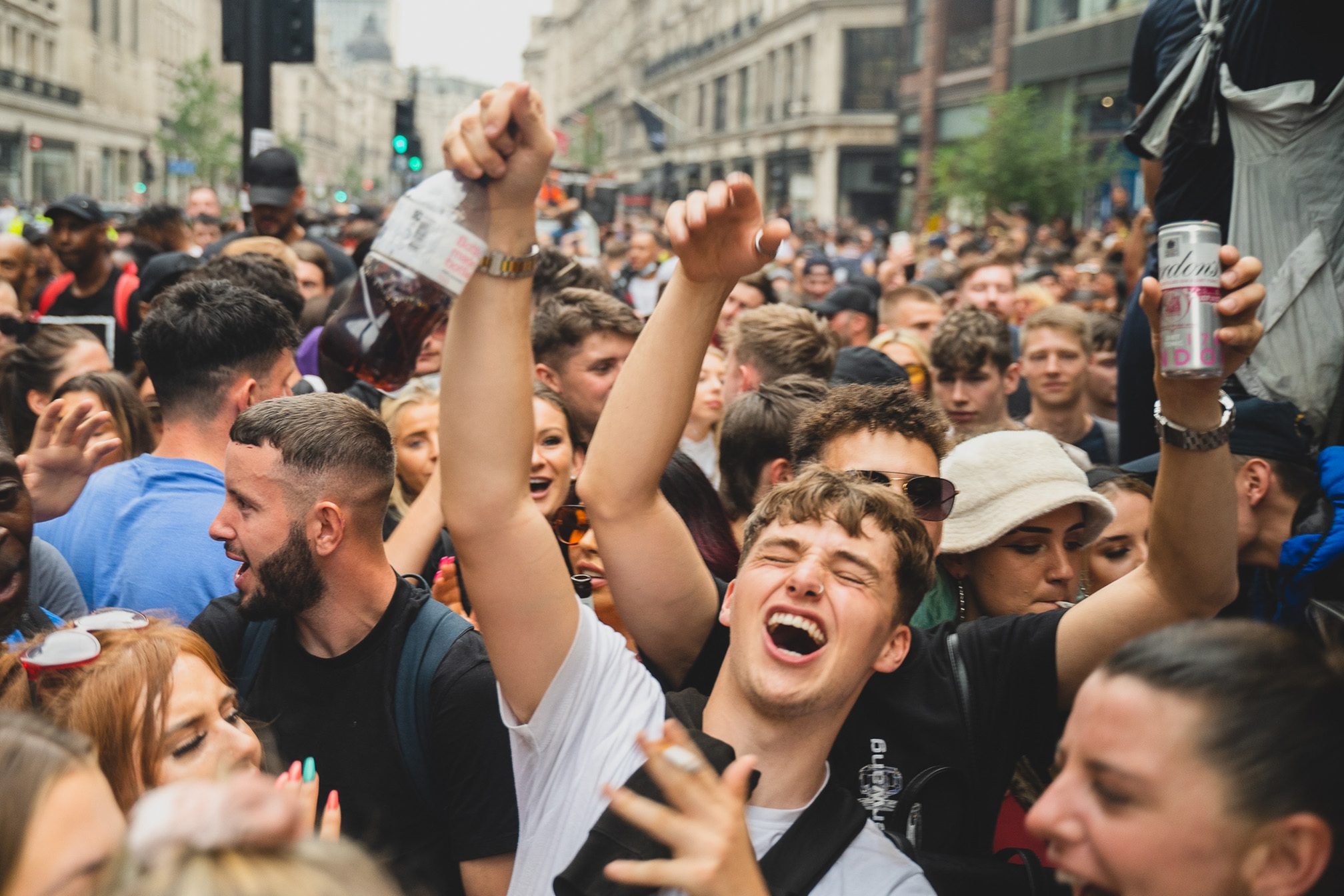The image captures a lively daytime street party in a bustling city, packed with men and women, predominantly aged 20 to 30, enjoying themselves. Central to the scene is a teenage boy holding a bottle, possibly alcohol or soda, in his right hand and a cigarette in his left. His eyes are closed, he’s shouting and smiling, exuding joy. Surrounding him are hundreds, possibly thousands, of people, their expressions equally exuberant, with many holding up bottles and cans. The crowd is so dense that the sidewalks are hidden, replaced by a "sea of hands and heads." They are hemmed in by cream-colored, three-story buildings on either side. Green traffic lights hang in the background, and the absence of cars emphasizes the street's transformation into a pedestrian-only revelry zone. The festive atmosphere is highlighted by the varied appearances: men with mostly short brown hair, and women with diverse hair colors like blonde, brown, and red, some wearing sunglasses on their heads.